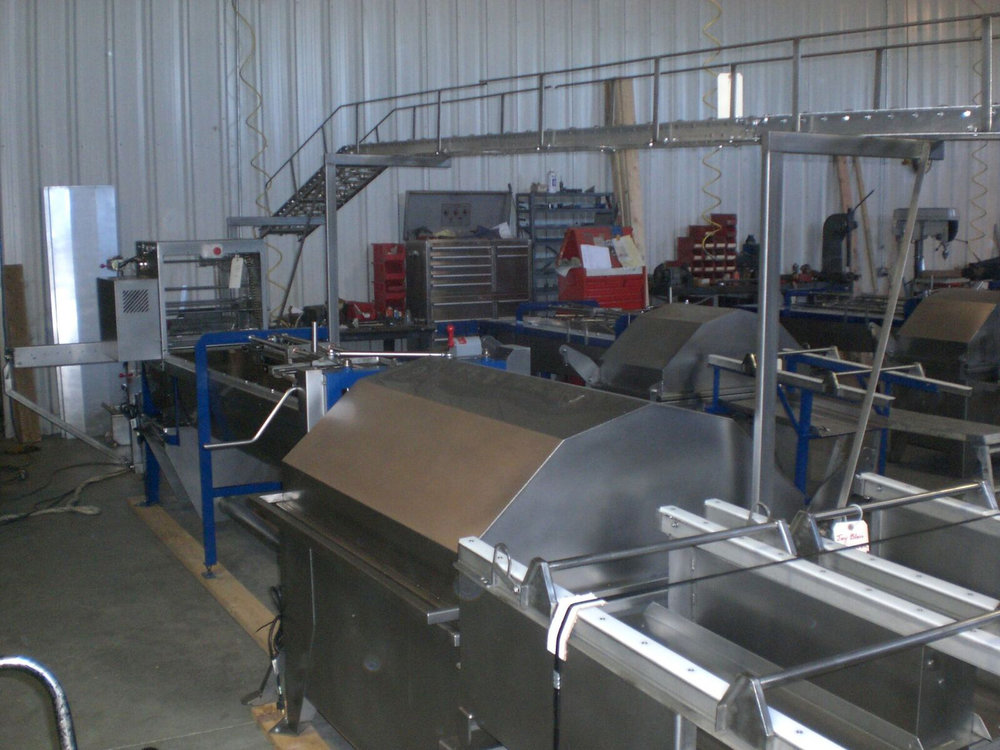This image captures the interior of a spacious warehouse, possibly repurposed as a large industrial kitchen or a storage facility for culinary equipment. The scene is dimly lit and appears amateurishly photographed, contributing to its raw industrial ambiance. Dominating the foreground is a massive stainless steel barbeque grill or grill-like apparatus, marked by a small tag. Adjacent to it, there are additional sizable heating and cooking elements, including components resembling troughs and spit-turning hot dog machines, all constructed from shiny metal, primarily stainless steel.

Beyond these cooking instruments, the midsection of the image showcases various other pieces of equipment, some painted bright blue and others potentially serving as conveyor belt systems, adding to the complexity and multifunctional nature of the space. Toolboxes and a drill press are visible at the back, underscoring the warehouse's utilitarian character. Overhead, spans a bridge or aluminum walkway, indicating a connected and navigable upper level, which hints at a structured organizational system. The walls, clad in vertically striped white metal panels, contribute to the pole barn-like aesthetic of this diverse equipment repository.